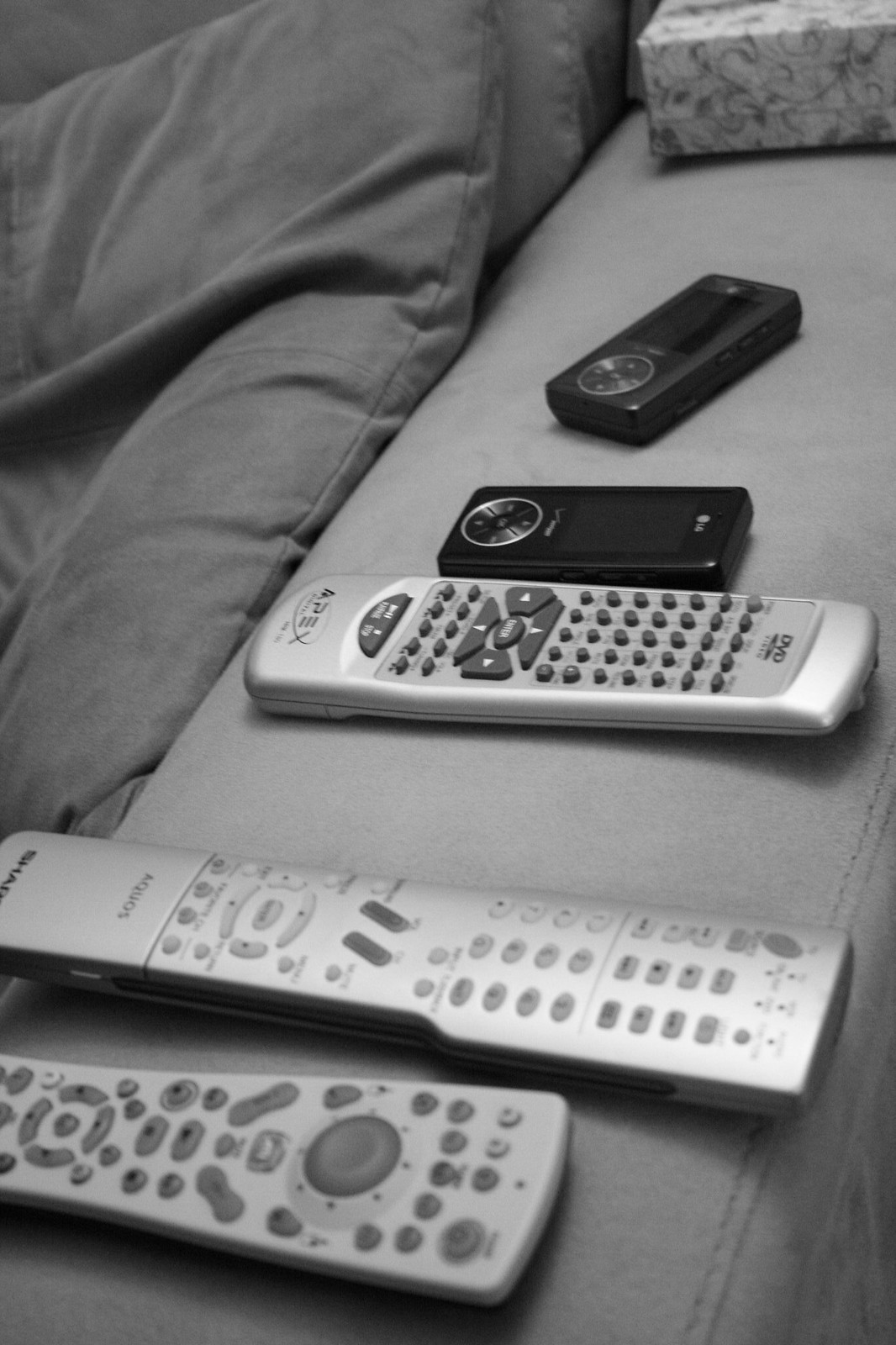The color photograph features a neatly aligned row of five remote controls and two smaller black electronic devices, possibly old-style flip phones, all resting on the wide, squared arm of a gray micro-suede couch. The remotes are predominantly silver with variously colored buttons—gray, white, and black. Their labels include kanji characters, and one is marked "Sharp Aqueous." The photo highlights a grayscale palette, with the couch, wrinkled gray pillow, and background contributing to the monochromatic theme. Shadows cast by the devices add depth to the composition. A black and white variegated item and the edge of a puffy suede cushion in the background, along with the glimpse of a Kleenex box, provide additional context to the indoor setting.